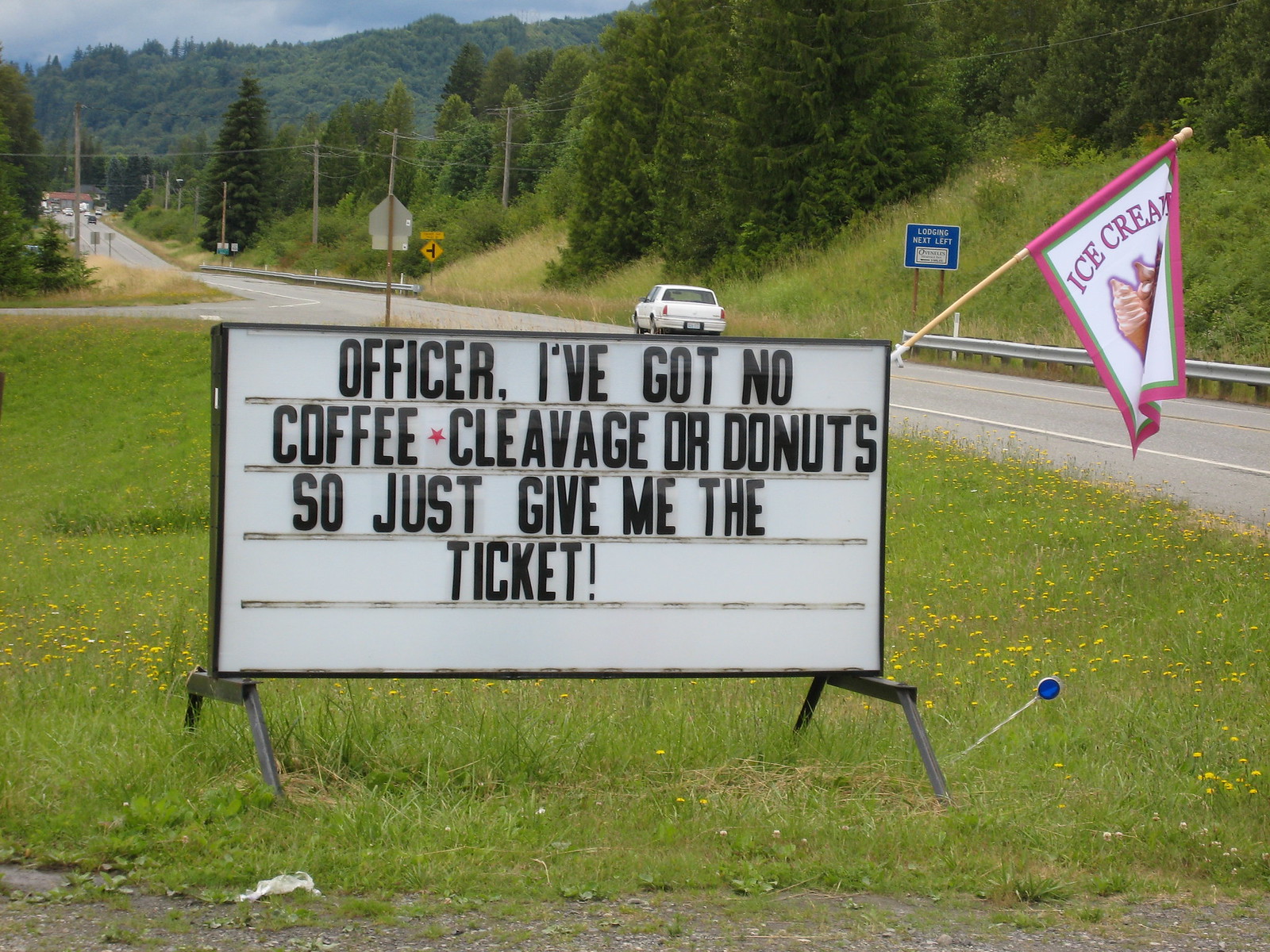This image shows a vibrant scene along a road, featuring a prominent white rectangular sign supported by four bars. The sign has a thin black border and large black text that humorously reads, "Officer, I've got no coffee, cleavage, or donuts, so just give me the ticket!" punctuated by an exclamation mark and adorned with a small red star. Hanging from the top right corner of the sign is a wooden pole with a red flag, which has the word "ice cream" written in red text on a white rectangle background alongside an image of an ice cream cone. In the bottom right corner, a blue lollipop is visible, sticking out from the grassy area below the sign. The area is lush with green grass and scattered yellow daisies, set against a picturesque backdrop of a mountain range. A long road stretches into the distance with telephone poles and tall pine trees lining it. On this road, a white car passes by, heading towards a town in the distance.